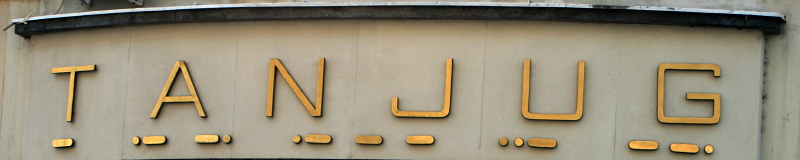This photograph features a sign on a building, likely an office structure. The sign displays the name "TANJUG" in prominent golden letters. The background of the sign is a tannish concrete wall, contributing to a modern yet industrial aesthetic. Beneath each letter of "TANJUG," there are unique oblong shapes, resembling a series of dots and dashes suggestive of Morse code. Although the exact meaning of these shapes is unclear, they add an intriguing, cryptic detail to the sign. The rest of the building isn't visible in the photograph, keeping the focus solely on the Tanjug sign against the textured concrete surface.